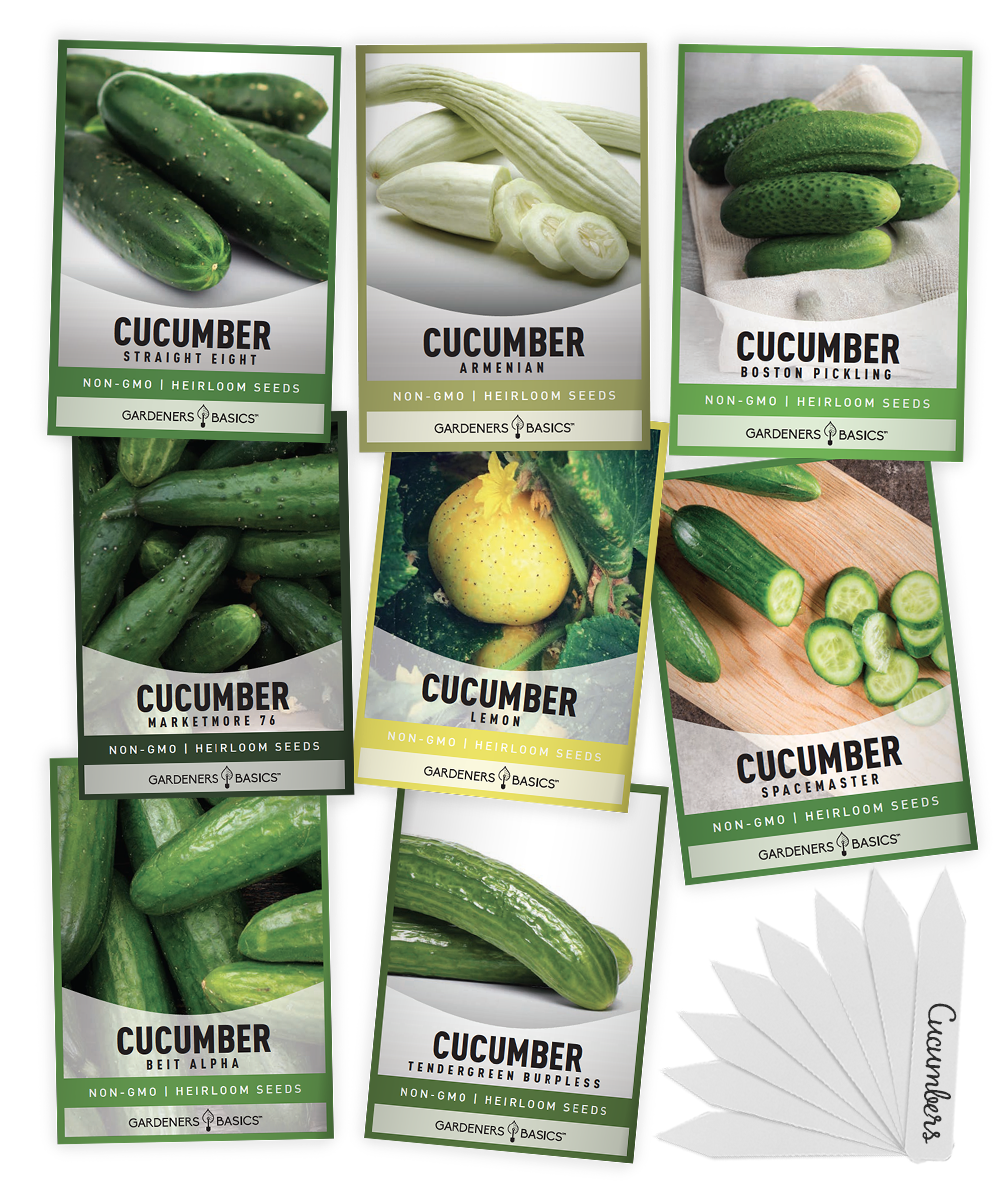The image showcases a variety of cucumber seed packets arranged in three rows. The top two rows each contain three packets, while the bottom row has two packets. Positioned to the right are several white garden picks, fanned out. The garden pick on the far right is labeled "cucumbers" in cursive black font. The seed packets are primarily from Gardner's Basics and feature different cucumber varieties. 

Starting from the top left, the first packet displays an image of cucumbers with the label "Cucumber Straight Eight" in black, followed by "non-GMO heirloom seeds" in white, and "Gardner's Basics" in black. To the right of it is "Cucumber Armenian," also from Gardner's Basics. Other varieties in the collection include "Boston Pickling," "Marketmore 76," "Lemon," "Space Master," "Bet Alpha," and "Tendergreen Burpless." Each packet represents different seeds perfect for planting cucumbers.